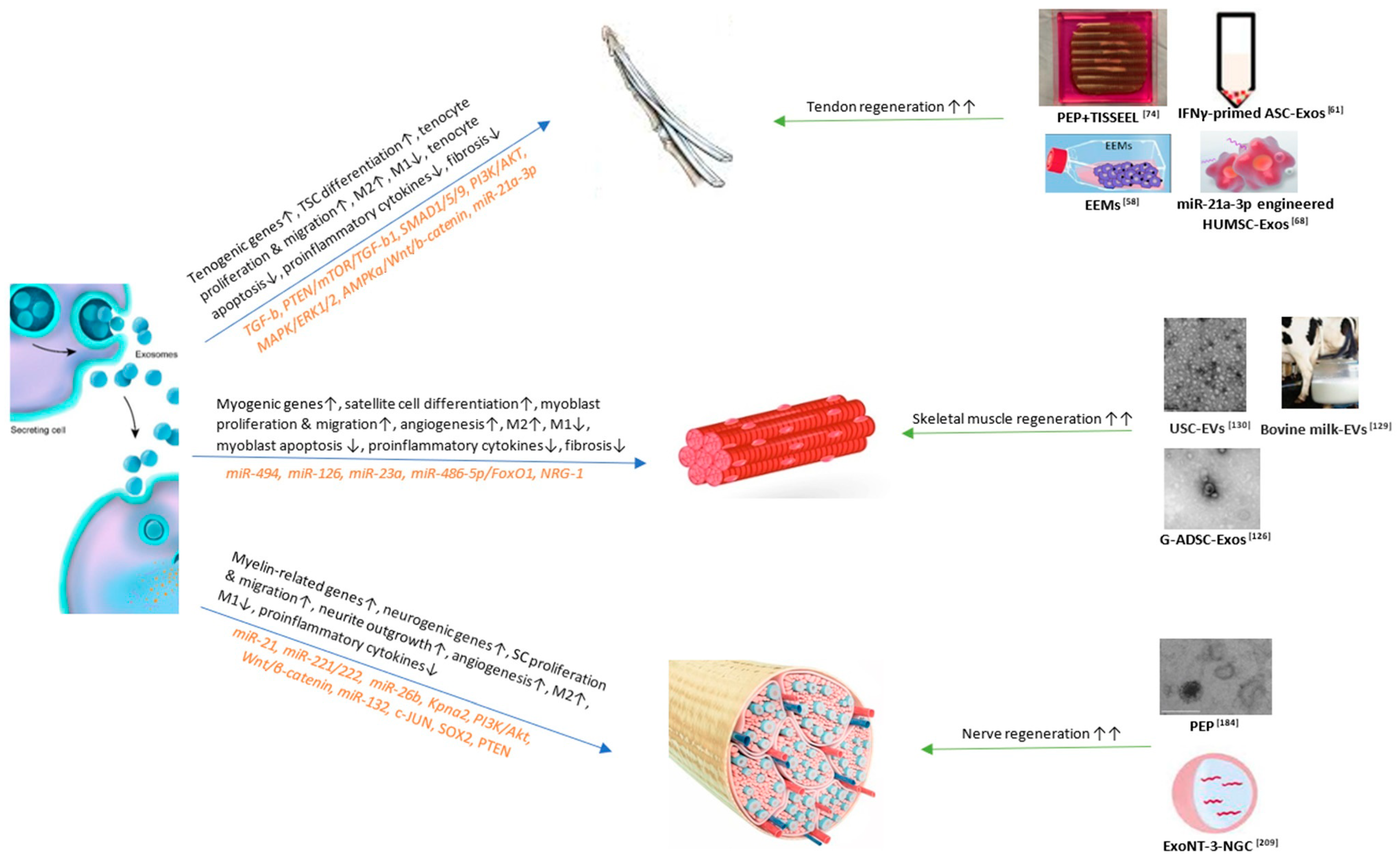This poster is an intricate flow chart detailing bio-inspired functional materials focused on cellular regeneration, including nerve, skeletal muscle, and tendon regeneration. Set against a white background, it features 14 distinct images that meticulously track the progression from one element to the next. At the top right, the poster showcases four images labeled PEP and various chemical compounds that illustrate the tendon regeneration process, including tenogenic genes, tendon stem cell (TSC) differentiation, tenocyte proliferation, and fibrosis. Below this, the skeletal muscle regeneration section is highlighted with three chemical compound images and an illustration of muscle fibers, explaining myogenic genes, satellite cell differentiation, and angiogenesis. Further down, the nerve regeneration area features two chemical compound images and a cross-sectional diagram of a nerve, detailing myelin-related genes, neurogenic genes, Schwann cell (SC) proliferation, and neurocyte outgrowth. The left-hand side of the poster graphically depicts cells, including a sequence where blue dots enter a purple cell, symbolizing cellular interaction. The central part of the poster presents red, spring-like muscle fibers and tendons, each accompanied by extensive text explaining the genetic relationships and cellular processes involved in regeneration. This scientifically dense and visually detailed poster provides a comprehensive overview of cellular regeneration pathways, invaluable for students and researchers in the field.